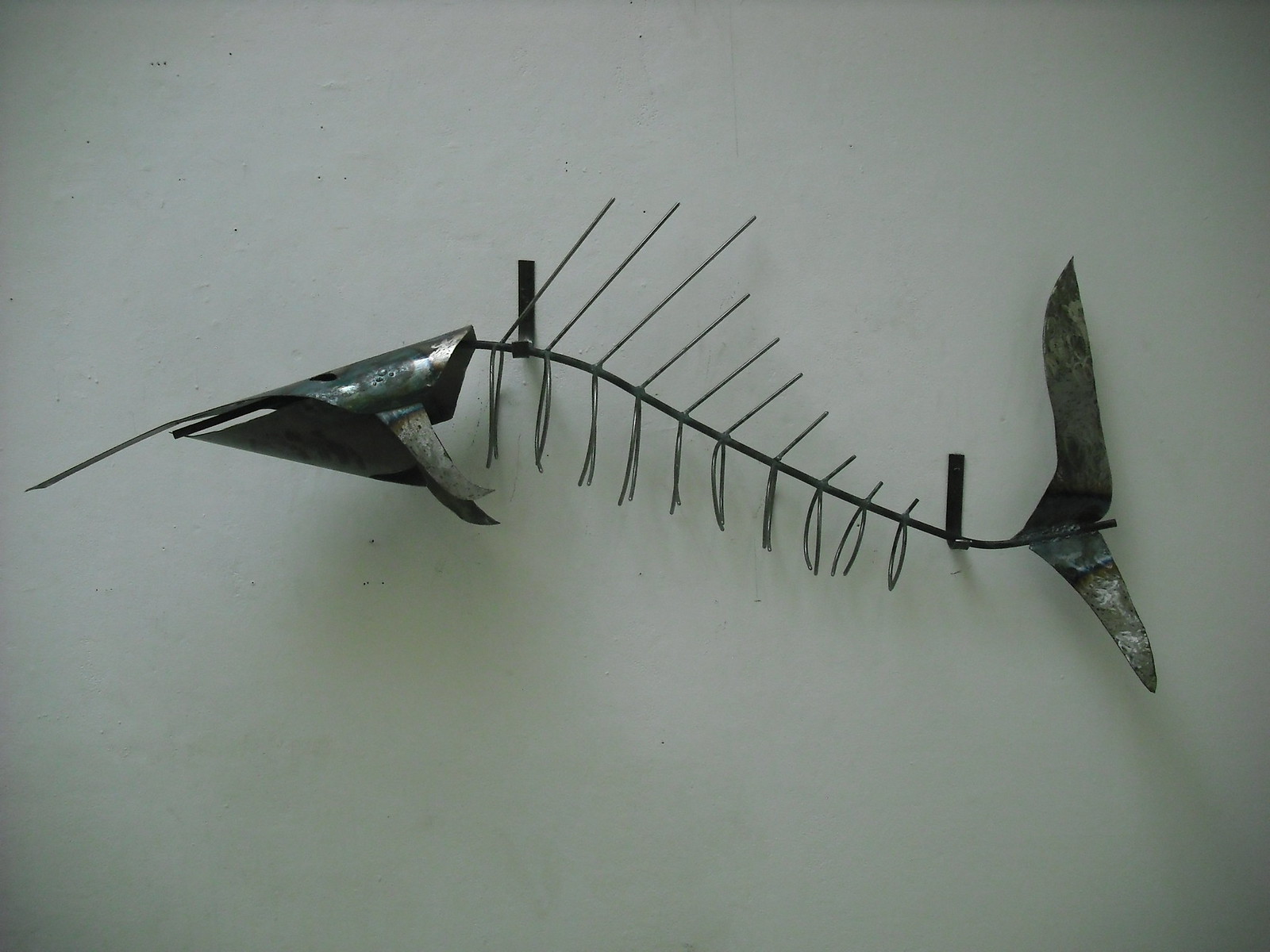The image depicts a detailed metal artwork resembling a fish skeleton, possibly a swordfish, mounted on a slightly grayish white plaster wall. The sculpture is suspended by two plain J-shaped hooks; the left hook is positioned slightly higher than the right. The fish, crafted from a black, almost shiny metal likely made of brass or copper, features a long pointy nose and a tail with two distinct fins— the top fin is vertically elongated, about twice the length of the downward-pointing bottom fin. The midsection reveals sparse, curved metal ribs, simulating a skeletal appearance. The spine, appearing as a thin, straight metal rod, connects the head to the tail, traversing a sequence of gradually shorter metal strips emerging from the spine to mimic the fish's decayed structure. The entire piece measures approximately five inches tall and six inches wide, artistically capturing the essence of a fish reduced to its skeletal framework.